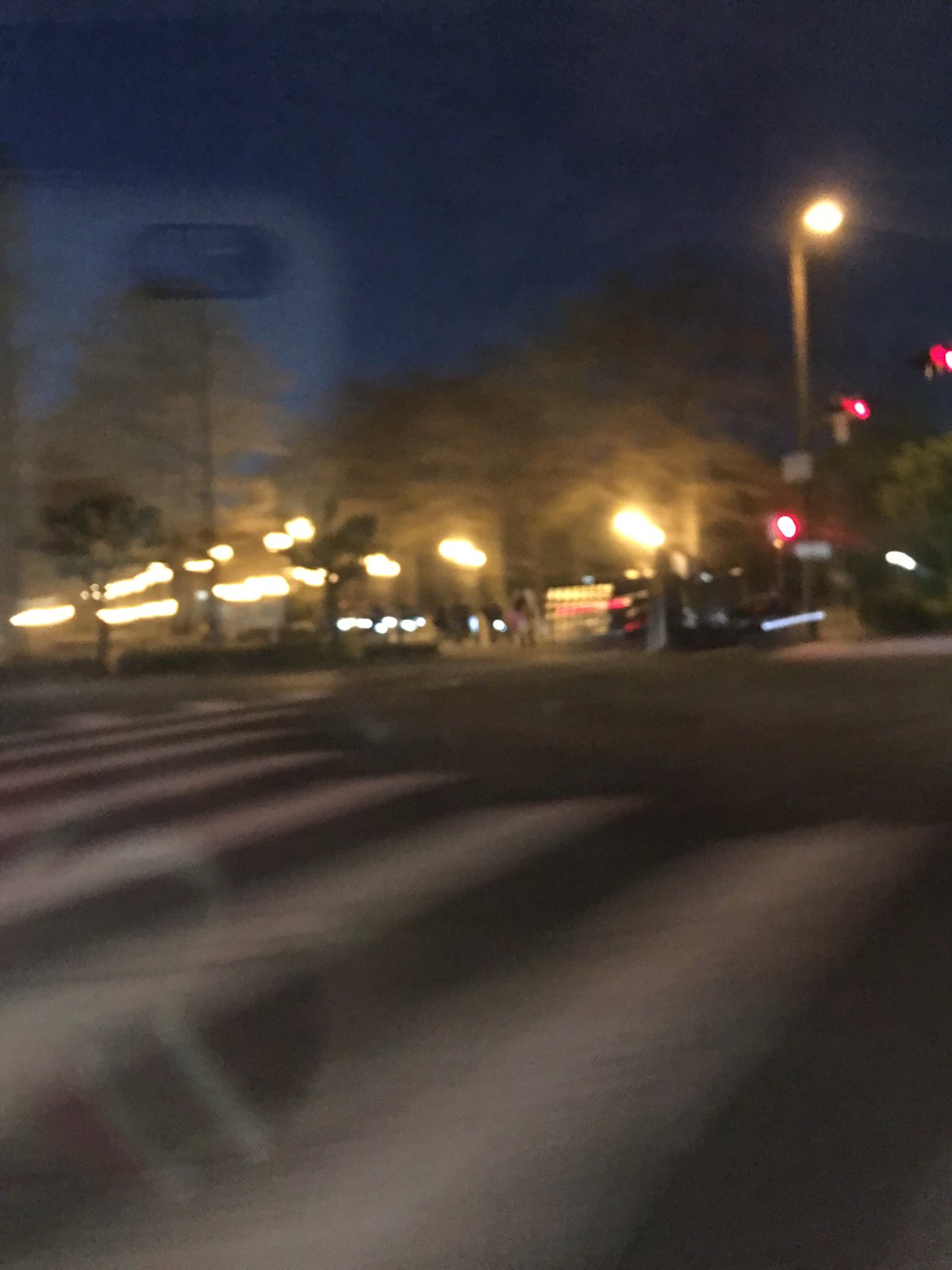A blurry photograph, taken with a phone in a white case through a moving car window, captures the vibrant essence of a busy street. The reflection of the phone is visible in the top left corner, affirming the assumption that the image was snapped from inside a moving vehicle. The main focus of the picture is a crosswalk with large, distinct white lines extending across the road, which the car is currently traversing. In the background, towering trees almost match the height of a prominent, stadium-like streetlamp, creating an imposing silhouette against the sky. Smaller streetlamps, blurred due to the car's motion, can be seen scattered around the scene. On the right-hand side, two traffic lights are captured, both glowing red, adding a vibrant contrast to the greenery and urban setup.